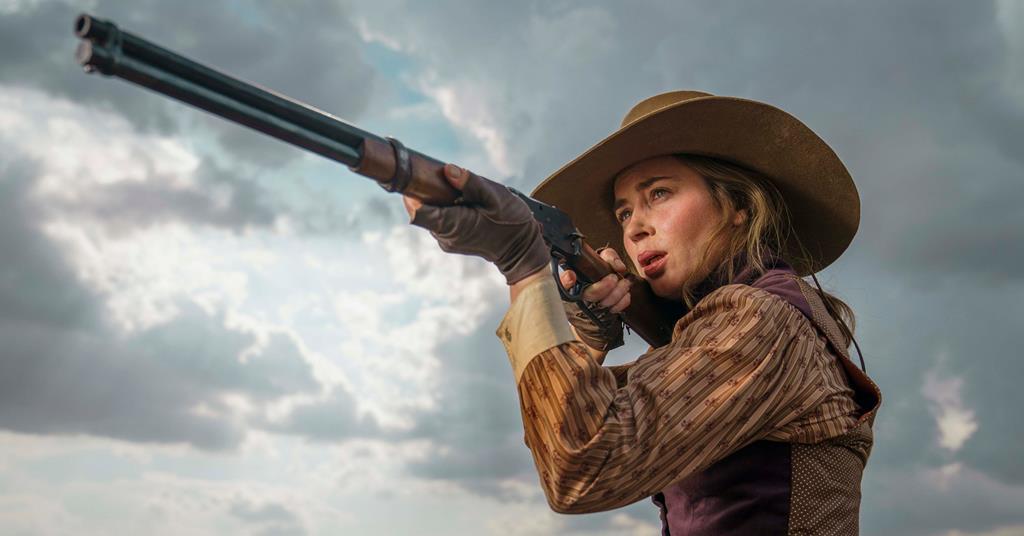A photograph captures a young blonde woman in Western-style clothing, slightly off-center to the right, aiming a long-barrel rifle with a serious and concentrated expression. She wears a brown cowboy hat and fingerless brown leather gloves. Her attire includes a long-sleeved floral shirt with vertical stripes and white cuffs, underneath a brown and tan vest with hints of purple and small white polka dots on the back. The rifle she holds is brown and black in color, with the grip and handle in brown and the barrel in black. The background is dominated by a cloudy sky, with streaks of gray and some blue peeking through. She gazes intently into the distance over the rifle's barrel, with her mouth slightly ajar, suggesting a moment of high tension. The image is framed from the waist up, emphasizing her poised stance and the looming overcast sky.